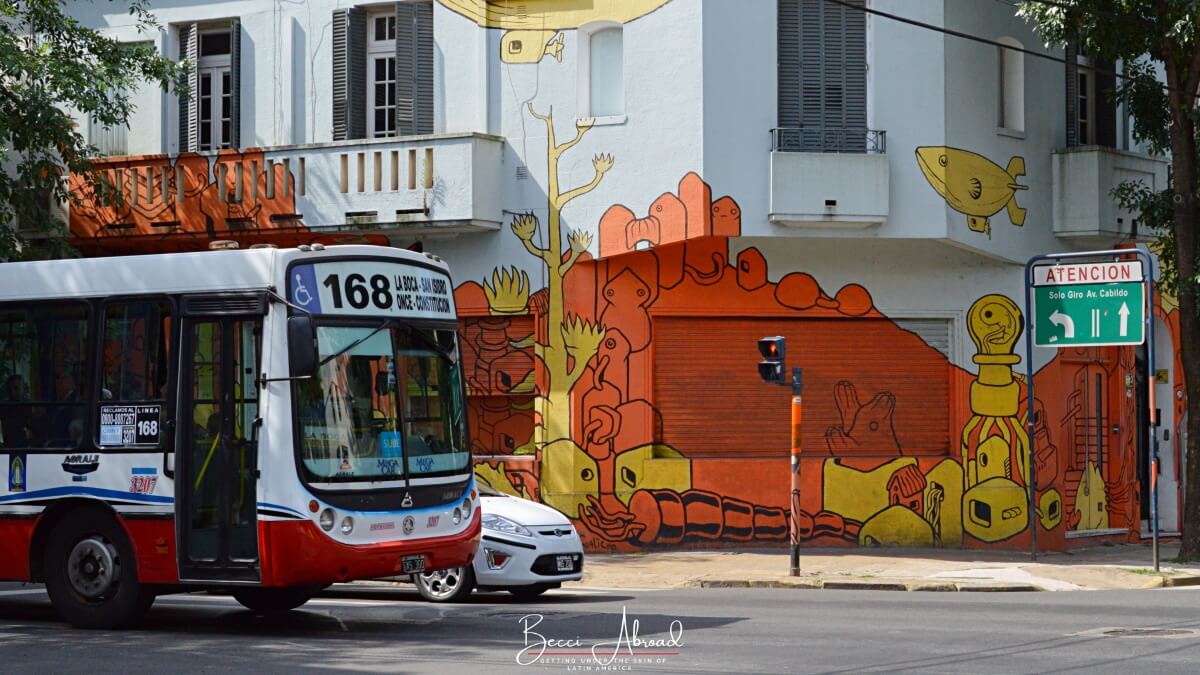This image depicts a bustling city street in Mexico, as indicated by a street sign on the right that reads "Atención" in Spanish. Dominating the background is a white apartment building adorned with vibrant red, orange, and yellow artwork. The mural features various whimsical objects, including block-like drawings, a fish-shaped blimp, and a three-legged robot. A small white car and a large city bus marked with the number 168 are traveling from left to right on the street below. The scene is set on a sunny day, with trees lining the urban downtown setting, adding to the lively atmosphere.